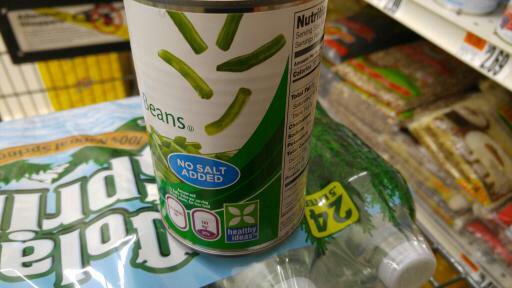In a grocery store aisle, a photo captures a shopping basket prominently in the foreground. Centered in the image is a can of green beans sitting atop a package of 24 bottled waters. The can features a white label with five neatly arranged green beans and the words "no salt added" in a blue circle, along with partial nutritional facts. The water package has a blue front with white lettering and displays a yellow square labeled "24." The clear bottles have white caps. Behind the basket, shelves are visible, stocked with various products. The bottom shelf seems to hold packages of rice, while the top shelf shows parts of two cans. The scene includes a mix of colors, including green, blue, white, orange, yellow, brown, and red, adding to the vivid depiction of the supermarket setting.